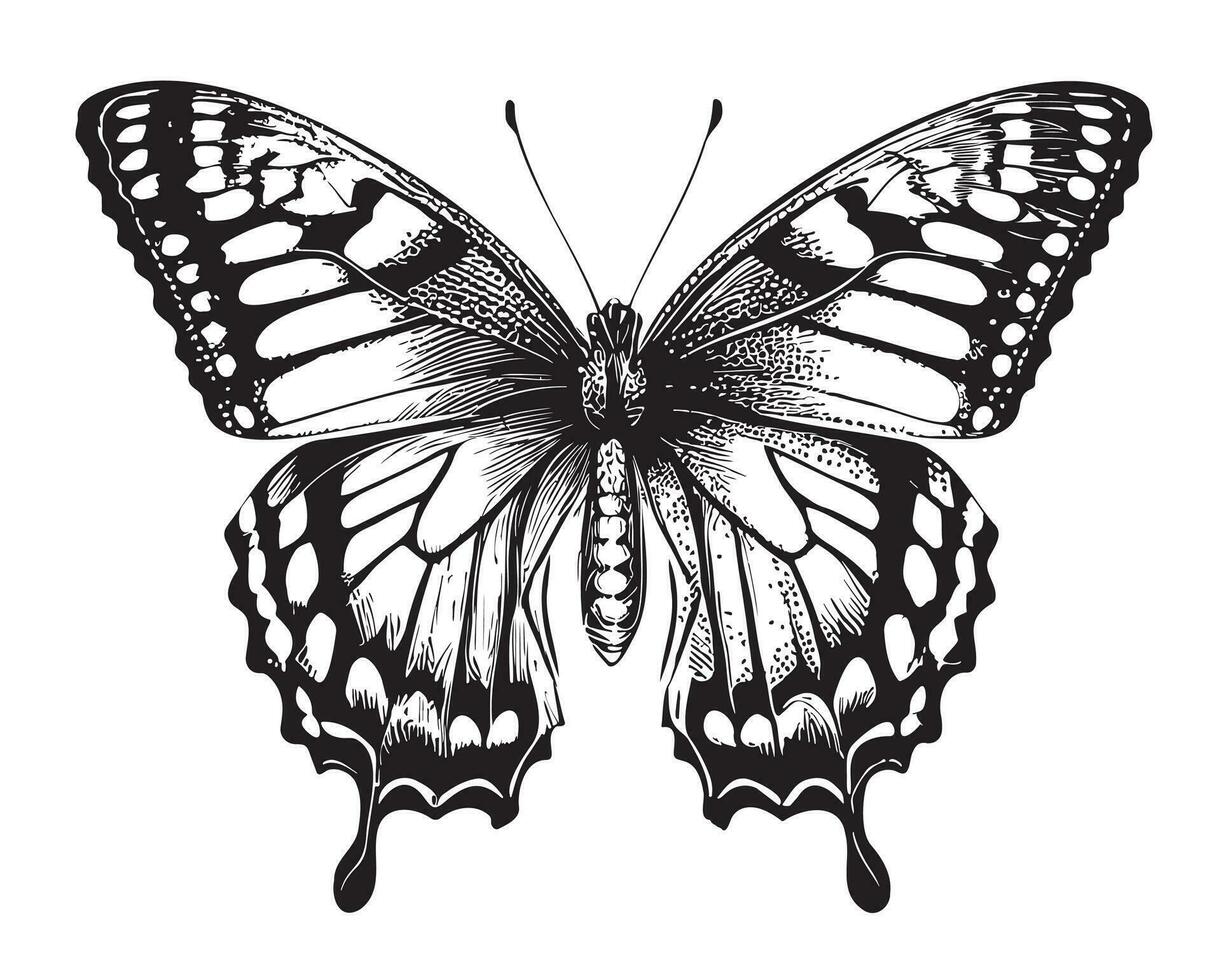This is a detailed black and white illustration of a butterfly, featuring the classic butterfly design with its wings spread out. The butterfly has two long antennas extending from its head, and a long body adorned with white dots. The wings are notably large, with the top wings shaped like triangles and the bottom wings more rounded, each incorporating teardrop-like designs. The image, reminiscent of a monarch butterfly, is composed entirely of shades of black, white, and gray, and is characterized by intricate dots and spots.